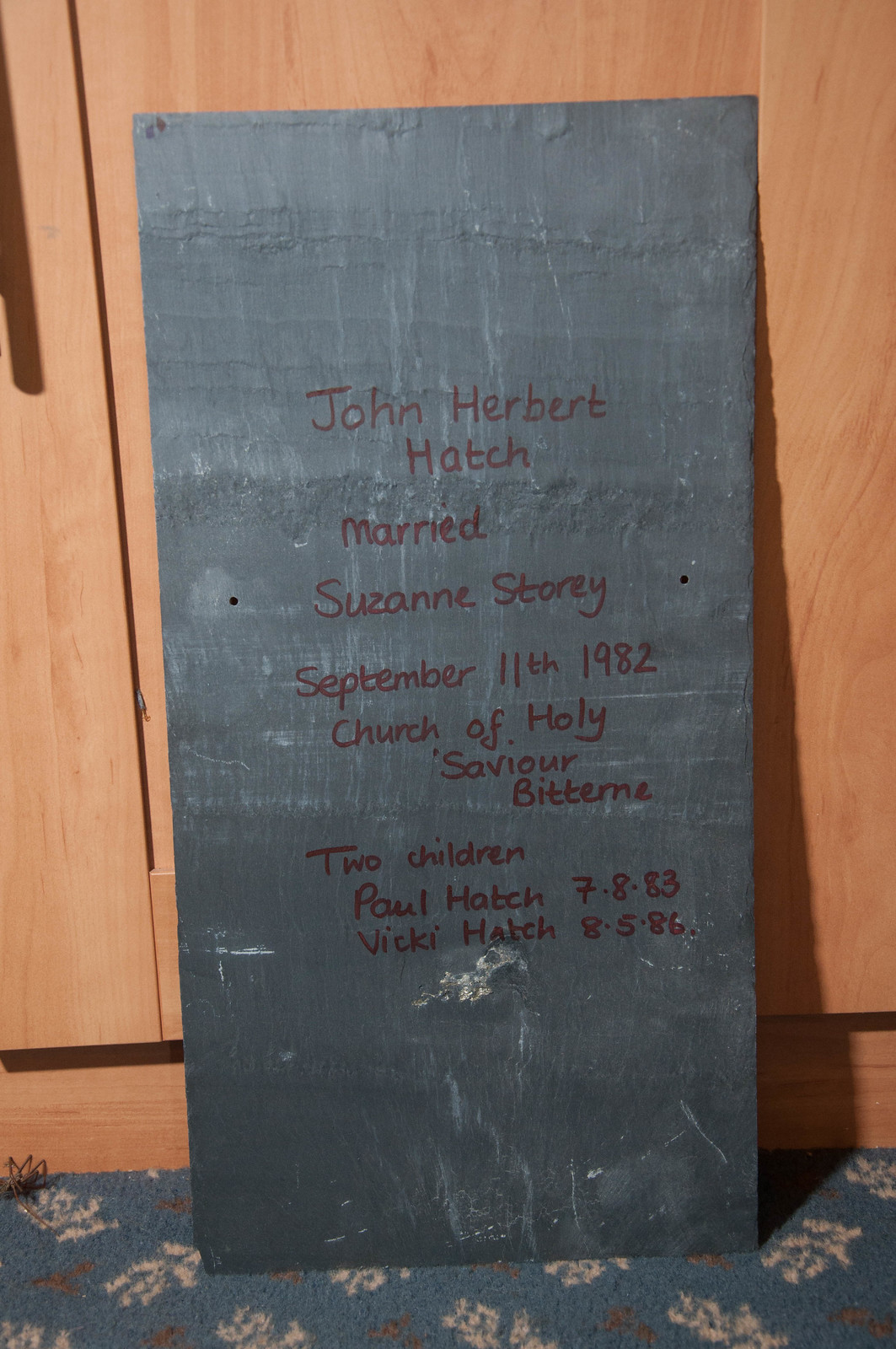This image features a photographic capture of a rectangular signboard leaning against a brown wooden door. The floor is adorned with a blue carpet featuring intricate brown, white, and red patterns. The dark green signboard stands out against this background. Inscribed in dark brown ink on the sign is a handwritten message detailing a family's history: "John Herbert Hatch married Susanna Story on September 11, 1982, at the Church of Holy Severe Paternity. They have two children: Paul Hatch (born July 8, 1983) and Vicky Hatch (born August 5, 1986)." The board also has a grey border with subtle hints of white.